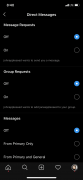A highly pixelated and blurry screenshot of an application in dark mode, featuring predominantly white text that is difficult to decipher. The image appears to be of a settings page, with multiple toggle switches labeled on and off. Some of the toggle sections seem to be related to device and fingerprint settings, though the text remains largely unreadable. Sporadic blue elements throughout the image resemble play buttons. At the bottom of the screenshot, there are various tabs, including icons for home, search, and profile, indicating that a user is signed in. The top of the image shows a fully charged battery and strong cell reception. The extreme blurriness suggests a lack of clarity, almost as if the details were intentionally obscured.